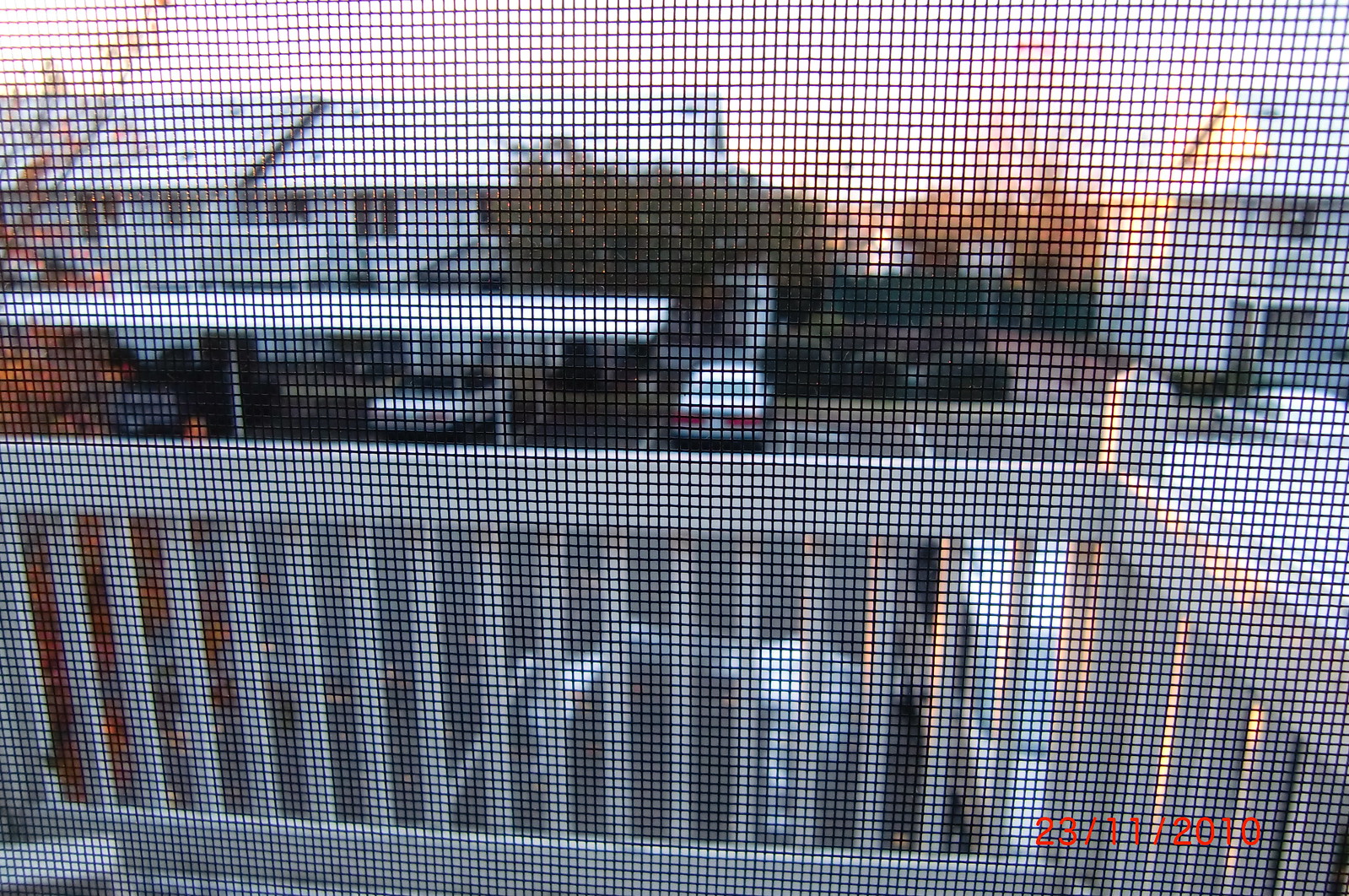The photograph appears to have been taken from within an apartment through a window or screen door, leading out onto a small balcony. The screen, present in front of the door or window, dominates the entire image, giving it a textured overlay. Beyond the screen, there is a view of the apartment's white balcony railing, a section of a parking lot with several cars, and a cluster of additional white apartment buildings in the background. The scene is slightly blurred, particularly the parking lot and the distant buildings, suggesting a depth of field effect. Trees are visible among the buildings, adding a natural element to the urban setting. In the bottom right corner of the image, a red date stamp reads "23-11-2010," indicating the photograph was taken on November 23, 2010. The overall lighting suggests it is later in the afternoon on a clear day.